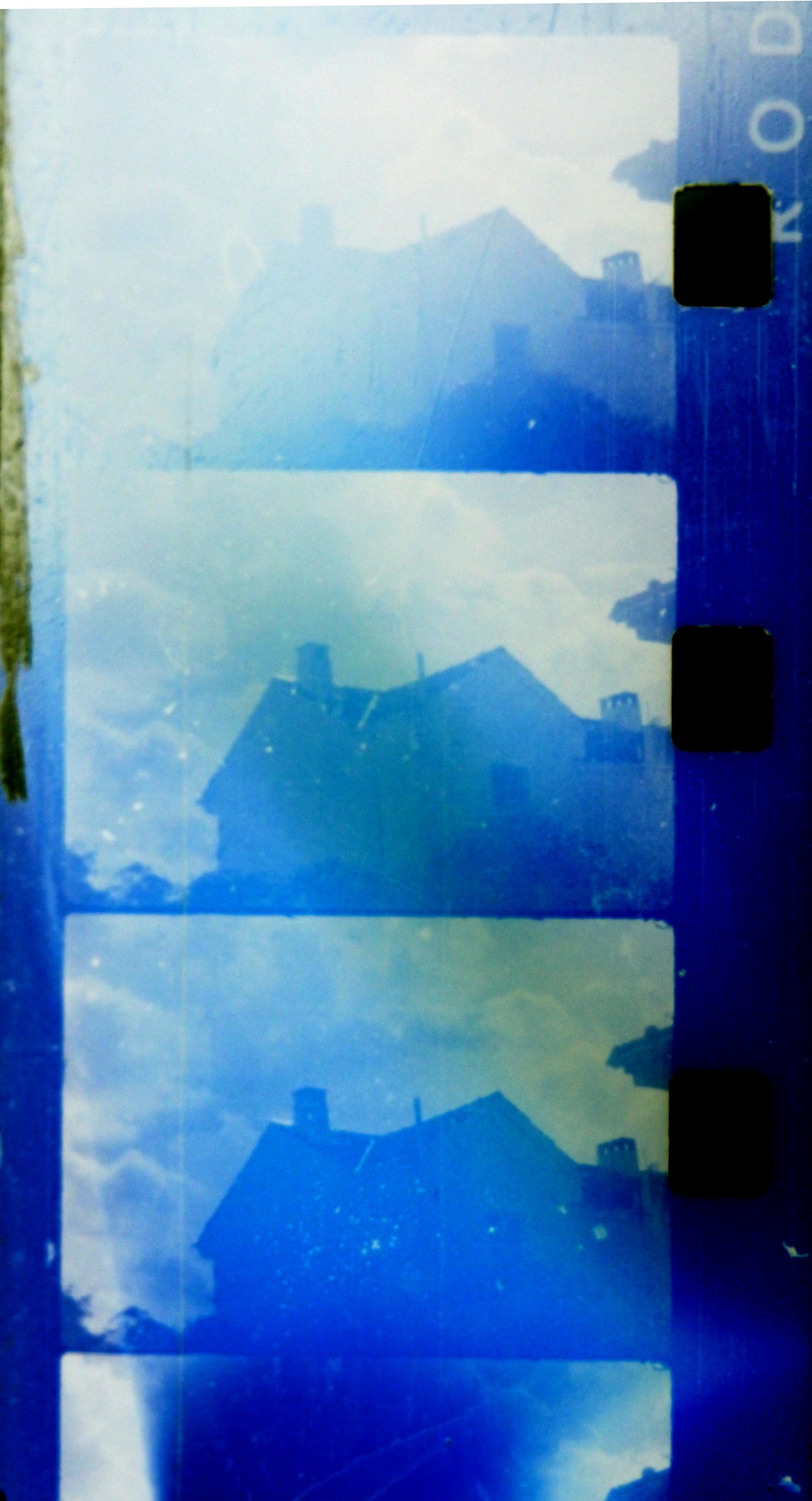This image appears to be a tattered and worn-out film negative, likely over 20 years old, depicting a series of images of a house. The overall color is a predominant blue, creating a hazy and blurry effect. There are three full images and a partial fourth one at the bottom, appearing as though it's cut off. The negative has notable black and white blotches scattered throughout. Significant black blotches are noticeable on the right-hand side, and there are black dots interspersed with blue areas along the side. The image retains characteristic elements of old 8mm film reels or traditional photography negatives, evoking a nostalgic sense of aged photographic processes.